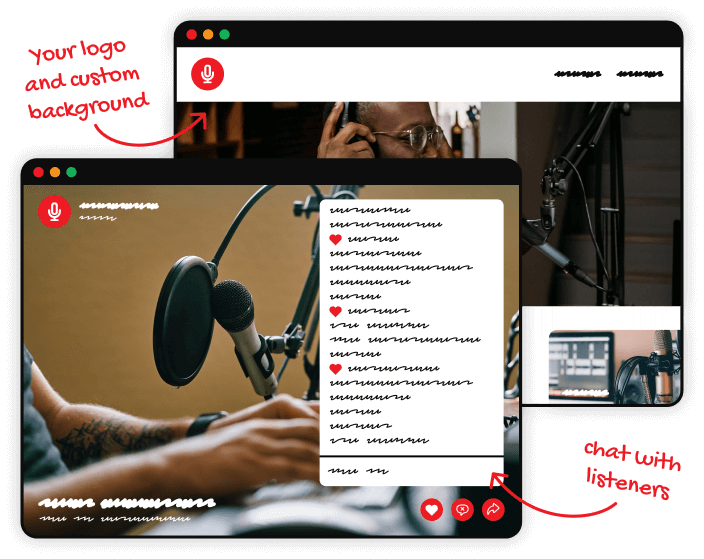This image features two overlaid browser windows on a white background. The primary browser window is situated at the top right of the image. Overlapping this, a second browser window is positioned at the bottom left, partially covering the first. Both browsers have black borders.

In the top left corner of the foreground browser, red text reads "Your logo and custom background." An arrow extends from the word "background" toward the top left corner of the background browser, indicating the customizable area.

In the bottom right corner of the foreground browser, the text "Chat with listeners" is visible, with an arrow pointing to the chat box located on the right side of the background browser.

The primary browser at the top right features a red microphone icon at the top of its window, with black text to its left. The overlapping browser at the bottom left also has a red microphone icon at its top left corner and a prominent chat box to the right.